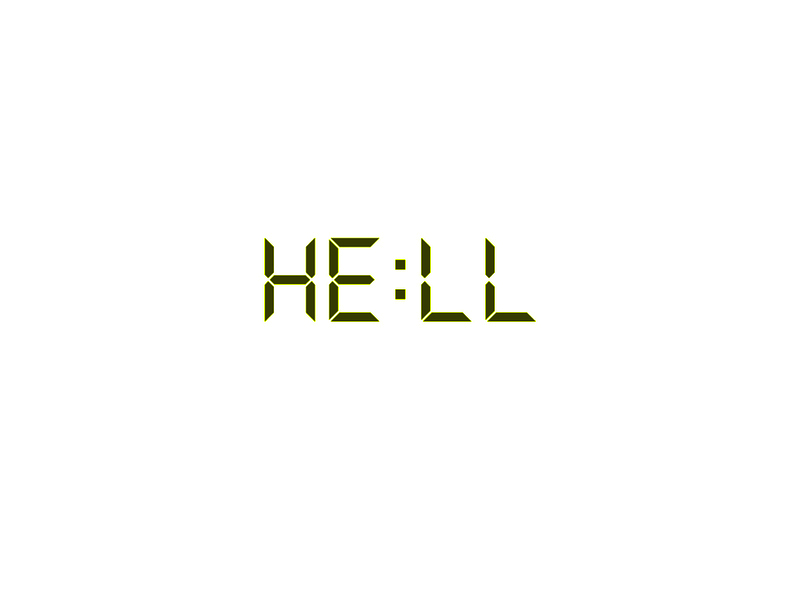The image depicts a basic white background featuring green digital-like text, reminiscent of an LCD display commonly found on calculators, clocks, or old cell phones. The text spells out "H-E : L-L," intended to mimic the word "hell" when digits on a calculator are flipped upside down. However, traditionally, the digits 7734 are used for this trick. The letters are in an olive green color, designed with spaces and pointed tips, characteristic of classic digital fonts. Despite a capital 'H' breaking the usual formatting, the image evokes a nostalgic reference to the calculator wordplay.